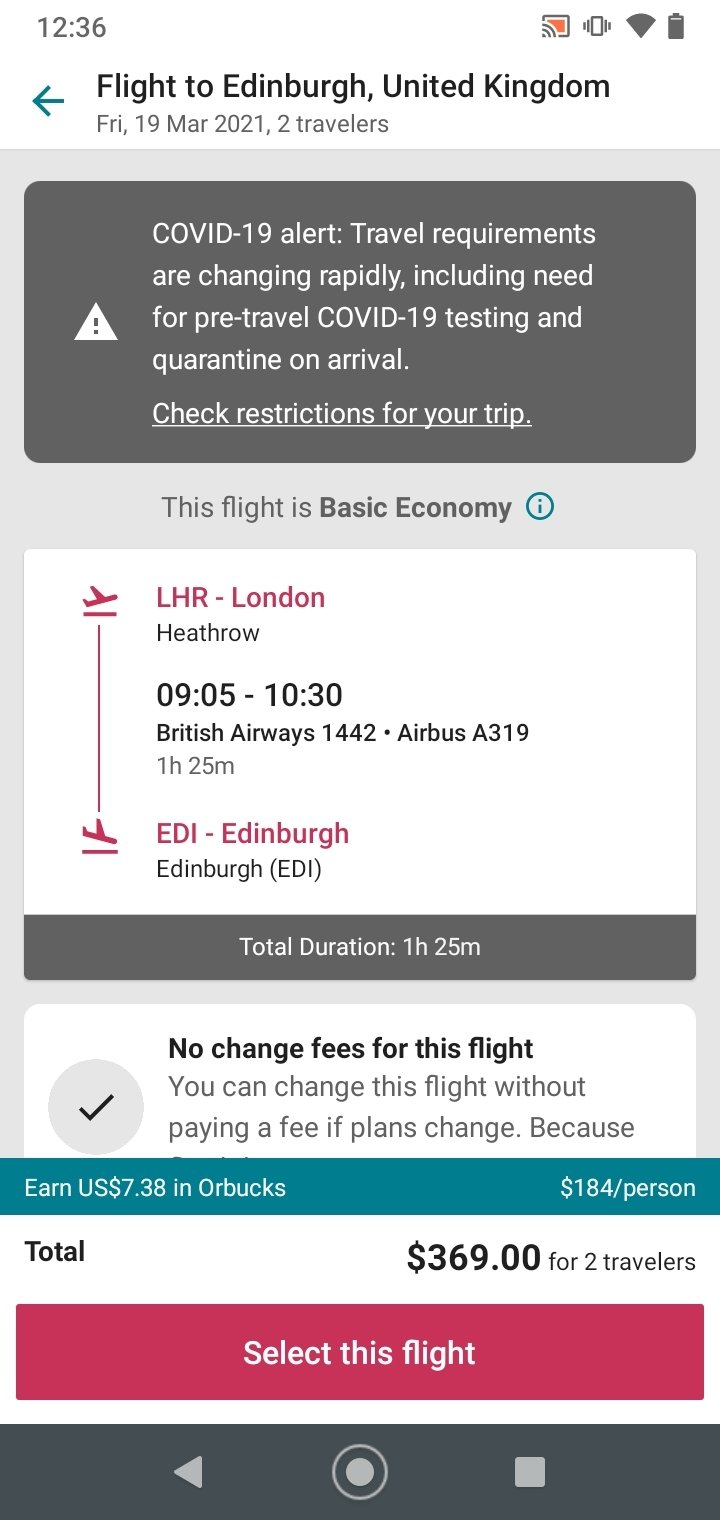Here we have a detailed breakdown of a flight from London to Edinburgh, United Kingdom. 

The total flight duration is approximately 1 hour and 25 minutes. The cost for two travelers is $369, which averages to $184.50 per person. This particular flight offers a basic economy fare. 

The time displayed on the person's phone screen is 12:36 PM. A prominent reddish-pink button labeled "Select This Flight" is also visible, guiding users to book this flight option.